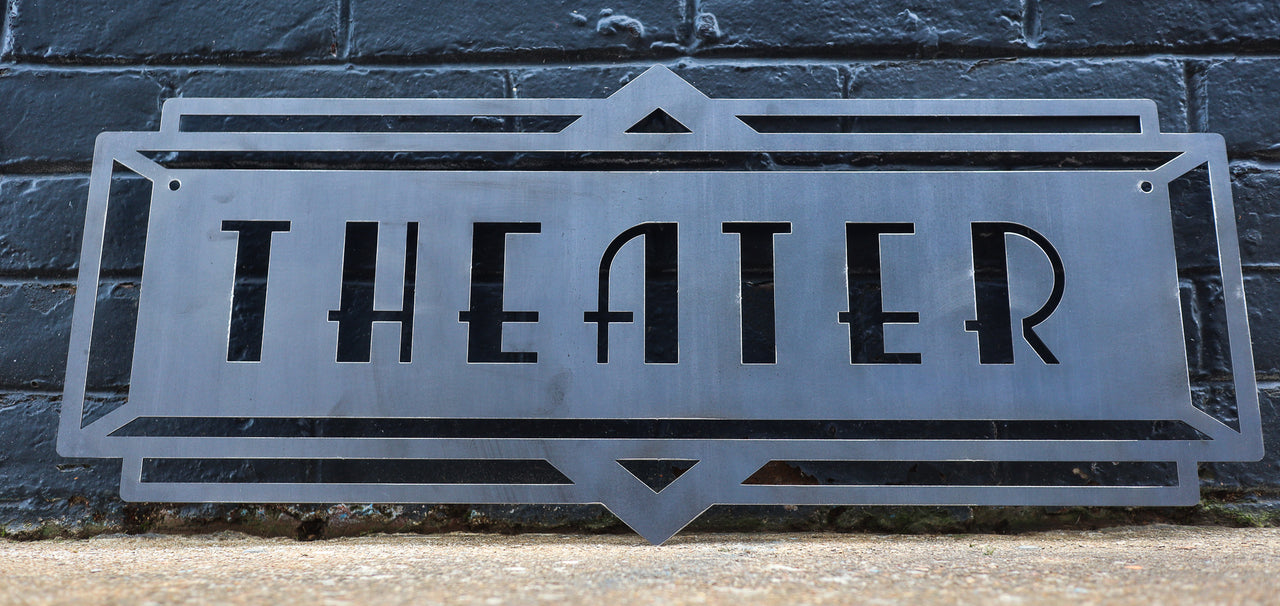This photographic image captures a sign of intricate design and Art Deco elegance, displayed outdoors against a gray-painted brick wall. The focal point is a rectangular silver metal plaque, prominently featuring the word "theater" in an Art Deco font. The sign, constructed from sturdy metal, is set within a metal frame that includes a decorative diamond cut-out on both the top and bottom.

The background of the text is a smooth, solid silver, adding to its sleek appearance. Around this central rectangle is a thin, silver border, which is further enhanced by a secondary, smaller border behind it. The outer frame is distinct with its diamond-shaped cut-outs—each diamond revealing an internal configuration consisting of a solid silver triangle paired with a black-centered triangle, placed at both the top and bottom of the plaque.

Adding depth to the scene, the image also features a light brown surface in the foreground, though it is unclear if this is attached to the wall or leaning against it. The wall itself reveals five rows of gray-painted bricks, providing a textured and neutral backdrop that highlights the elegant design of the sign. At the top corners of the plaque are two small eyelets, suggesting the mounting mechanism to the wall, completing this visually striking and finely detailed presentation of the word "theater."